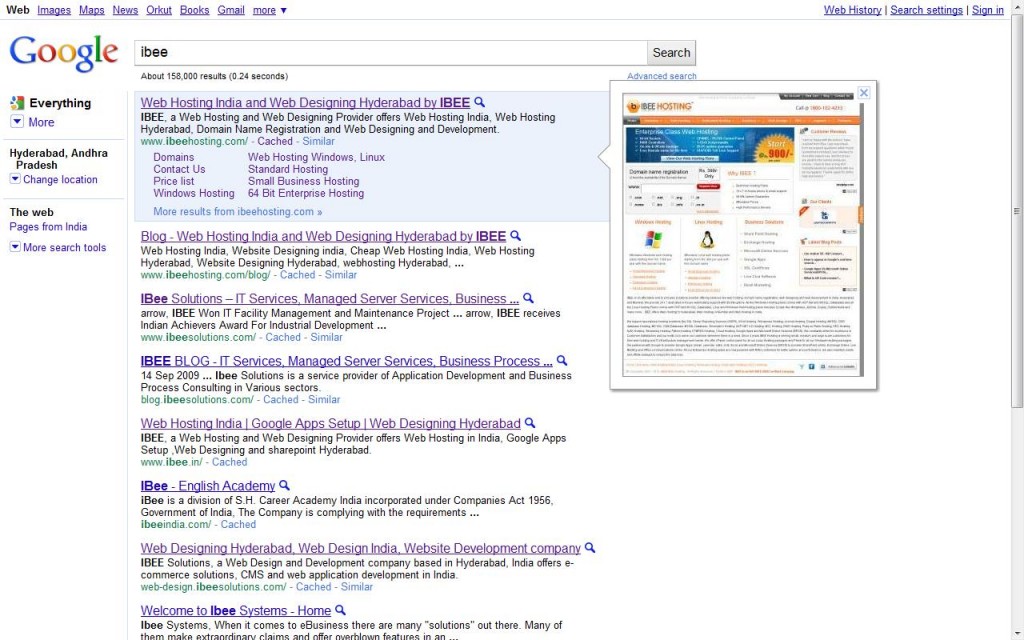The image captures a screenshot from the Google website interface. In the upper left-hand corner, the iconic Google logo is prominently displayed. Positioned above the logo is a navigational menu offering various clickable tabs: "Web," "Images," "Maps," "News," "Orkut," "Books," "Gmail," and a "More" tab with a downward arrow indicating additional options.

Adjacent to the logo is the familiar Google search bar. The search query entered here is "IBEE." Below this, the results indicate approximately 158,000 findings, retrieved in a brisk 0.24 seconds.

The search results start with a listing for "Web Hosting India and Web Designing Hyderabad by IBEE," providing a concise description stating, "IBEE is a web hosting and web design service provider, offering web hosting in India and Hyderabad, domain name registration, and web designing and development." Directly following this entry, there is a link to a blog titled "Web Hosting India and Web Designing Hyderabad by IBEE." Subsequent results include various IBEE-related sites, such as "IBEE Solutions" and an "IBEE blog," showcasing a range of IBEE websites and resources.